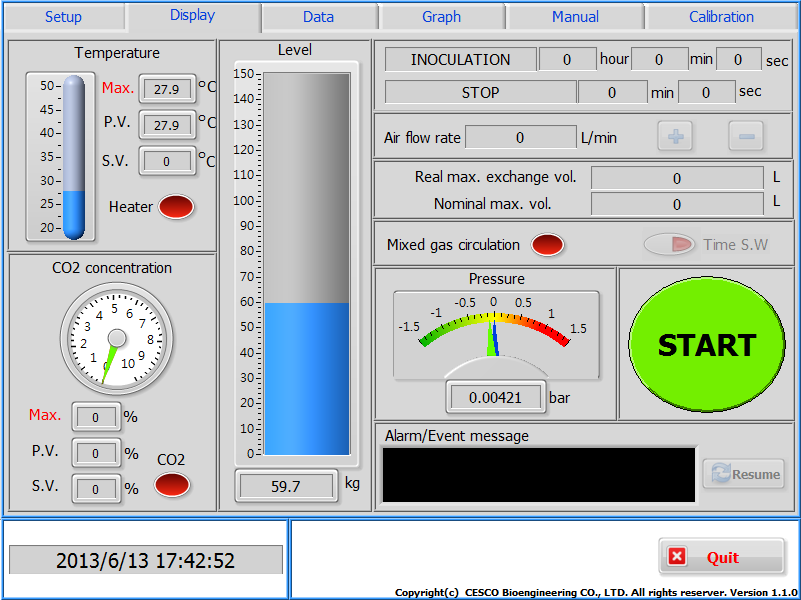The image displays the interface of a computerized system, likely related to environmental control or monitoring. At the top of the interface, there are six blue-text tabs labeled from left to right: Setup, Display, Data, Graph, Manual, and Calibration. The Display tab is currently selected. 

Below these tabs, the left-hand column features several tiles. The first tile is dedicated to Temperature, displaying a thermometer icon and readings labeled Max, PV (process value), and SV (set value). The Max and PV values are both 27.9, while the SV is zero. The thermometer graphic indicates a temperature between 25 and 30. The tile below this is for CO2 Concentration, featuring a circular dial meter currently at zero.

Adjacent to these tiles, in the right column, there is a section for Level indicating a current measurement of 59.7 kg. Further sections in this column include controls for Inoculation, Stop, and Air Flow Rate, along with a pressure gauge ranging from -1.5 to 1.5. An alarm and event message section is also present.

Additional details include a green start button, a date/time stamp of 2013-06-13 17:42:52, and a red X for quitting. The interface is copyrighted by Cisco Bioengineering Co. Ltd., Version 1.1.0.